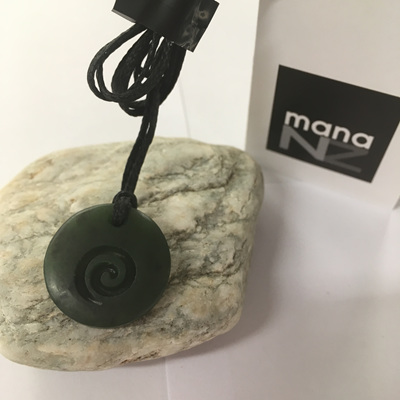The photo features a detailed image of a black circular pendant, resembling a medallion with a spiral design in its center, presumably made of stone. This pendant is attached to a black corded string and rests atop a light-colored rock. The setting is indoors, situated on a white tiled surface. In the top right corner of the image, there is a white bag displaying a black square with the text "MANA" in white letters, and "NZ" in gray letters beneath it, with the "N" in a slightly lighter shade of gray than the "Z."